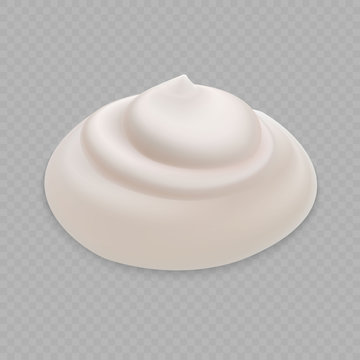The image showcases a white, semi-liquid dollop, resembling shaving cream, whipped cream, or a similar substance, positioned on a gray, semi-transparent background with a diamond-checkered pattern. This pile of cream forms a three-layered, swirling mound, broadening out at the base and tapering off to a rounded peak at the top. Slight drop shadows and subtle gradient shading provide a sense of dimension and form to the dollop, which occupies approximately 80% of the frame, emphasizing its circular, spread-out shape at the base, transitioning to a smaller, rounded tip. The overall layout is devoid of any other objects, text, or figures, focusing entirely on the intricately detailed cream against the patterned backdrop.